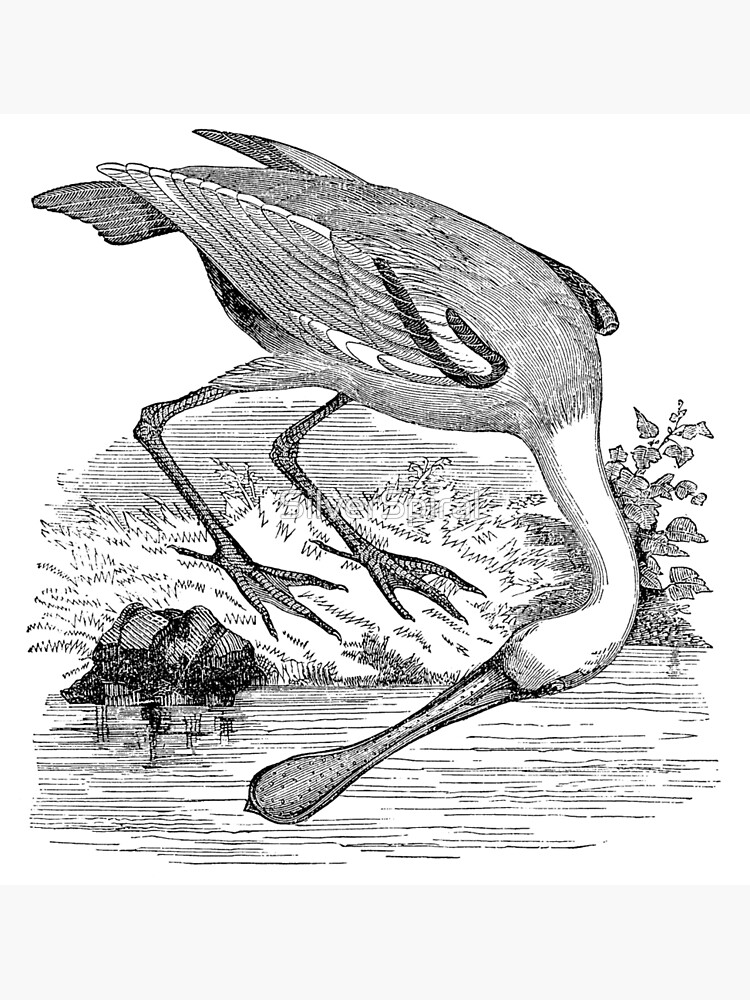This detailed black-and-white sketch, possibly created with pencil or thin black ink, portrays a bird with a long white neck, potentially a pelican or a duck-billed platypus. The bird, characterized by its substantial beak and detailed textures on its wings, stands on the grassy shore beside a lake or river. Its head is bent low, dipping into the water, likely in search of fish. The bird’s body, with darker shading for contrast and a meticulously rendered 3D effect, shows webbed feet with elongated toes and nails. The scene includes a nearby rock and additional realistic textures, including those of leaves in the background. The close-up perspective emphasizes the size and intricate detail of the bird and its surroundings.